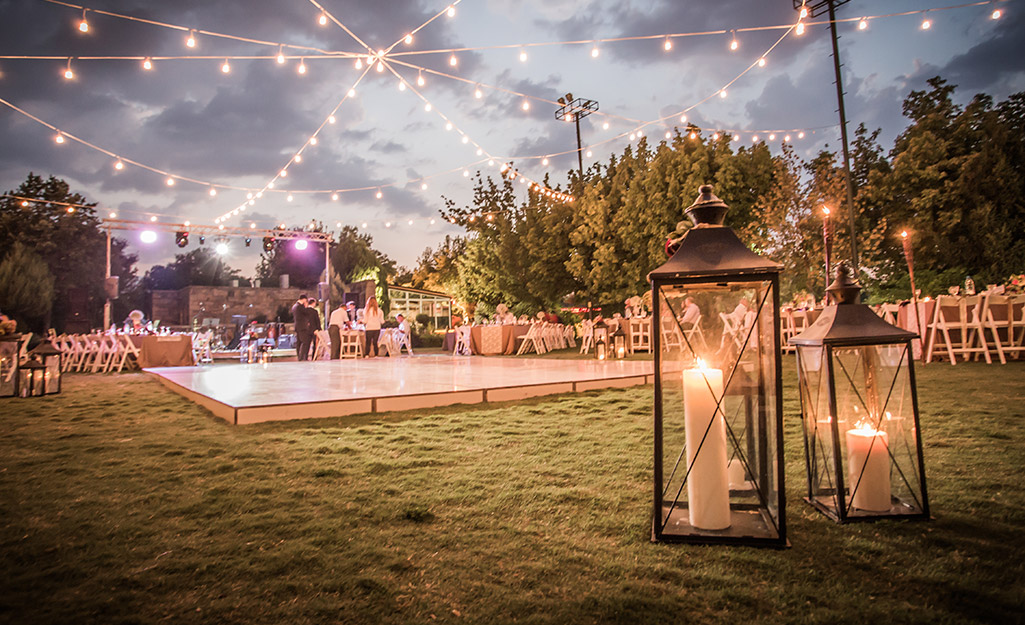The photograph depicts a large, lush green yard, seemingly set up for an outdoor event, possibly a wedding reception, during early evening. The sky above is overcast with gray clouds blending into a light grayish-blue hue. The ground is covered with meticulously short-cut grass, providing a verdant backdrop for the gathering.

At the center of the yard stands a large, square, raised white painted platform, most likely serving as the dance floor, with strings of globe lights converging overhead, attached to various black poles around the yard, creating a whimsical and festive atmosphere. Surrounding the dance floor, rows of folded white chairs are arranged, facing inward, suggesting an area set aside for guest seating.

In the bottom right corner of the image, there are two decorative, dark bronze-colored lanterns with glass sides, containing LED pillar lights that add a warm glow to the setting. Additional lanterns are placed towards the center-middle left side of the yard, further enhancing the ambiance. Mixed within the seating area, there are also white tables and more chairs, suggesting places for guests to dine and socialize amidst the enchanting outdoor scene. The backdrop includes an array of beautiful trees, contributing to the overall picturesque and serene environment of this likely celebratory event.